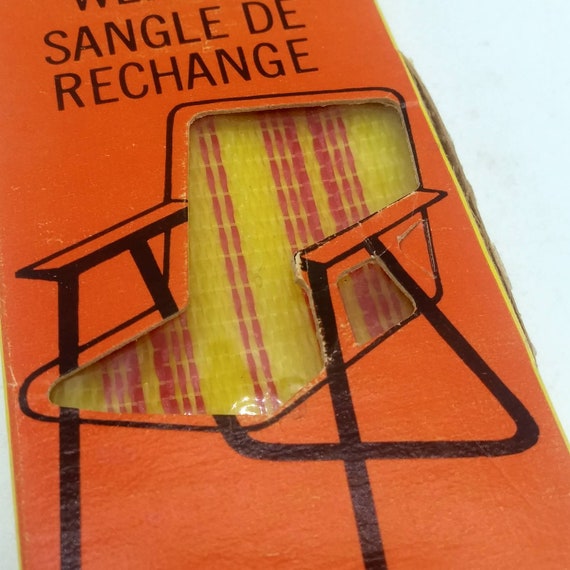The image appears to have been taken indoors and predominantly features an orange cardboard box with a white background on the right-hand side. The box has black lettering at the top that reads "SANGLE DE RECHANGE" and includes black dots on the edges of some letters. It appears to be a packaging for a lawn chair, which is depicted in an outline on the front of the box. The chair has a black iron frame with orange armrests and a cut-out area where the seating material is shown. The seat material itself is plasticky, woven in vibrant yellow and red stripes. The box is designed to give a peekaboo effect, displaying the colorful seating fabric through the cutout. The chair folds up, making it portable and convenient for storage.